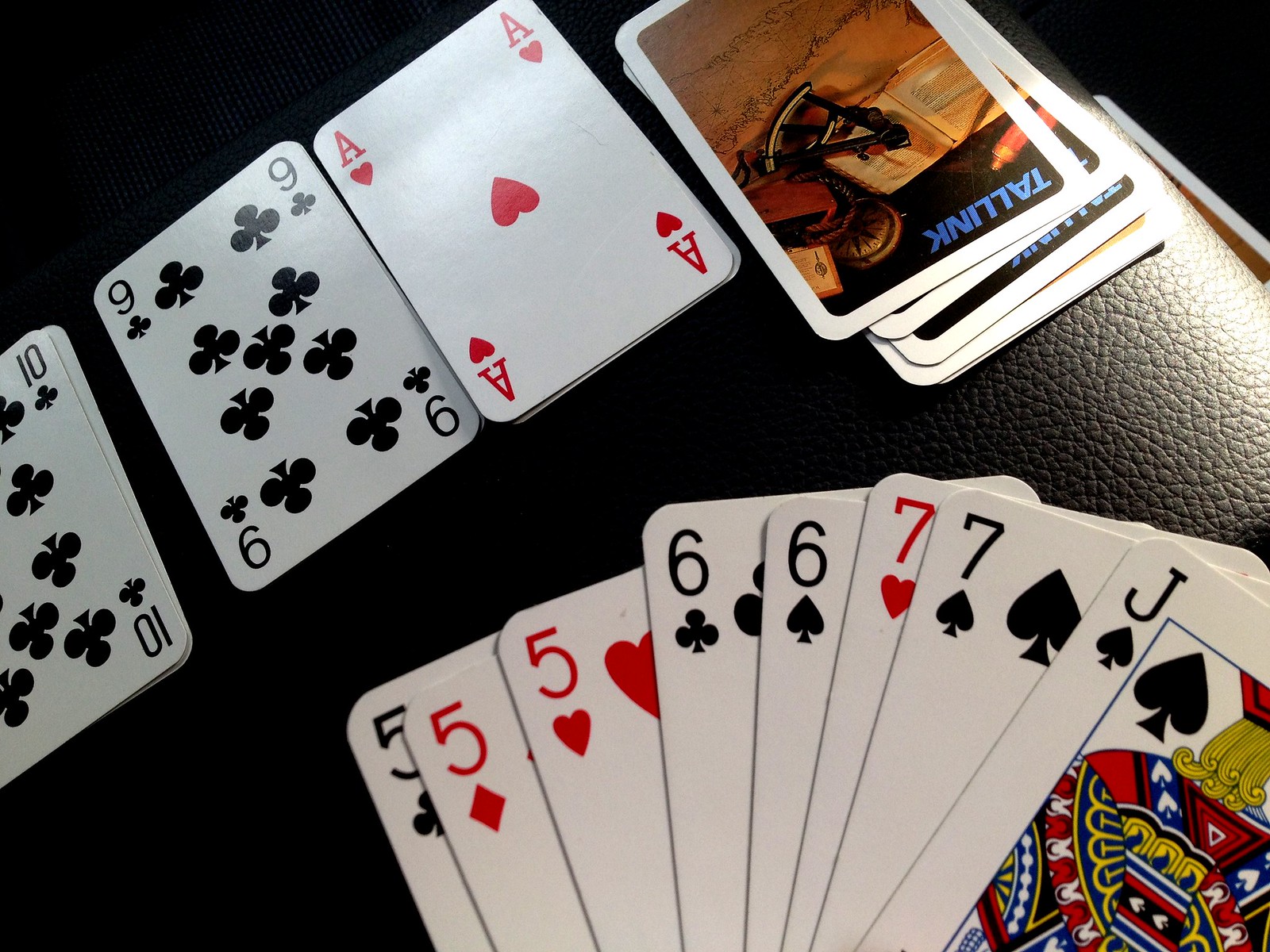The photograph features an array of playing cards set against a textured leather surface, highlighted by dramatic lighting that accentuates the indentations in the leather. At the top, the background transitions to a solid black, creating a stark contrast with the leather below. In the upper right corner of the image, a small stack of about five or six playing cards is neatly arranged face down. 

On the top left card of this pile, the text "T-A-L-L-I-N-K" is prominently displayed alongside an illustration of an open book. Spread out atop the leather, the cards are organized meticulously, starting from the top left with a sequence of white cards adorned with either black or red numbers and suits. The first row features a 10 of clubs (black), a 9 of clubs (black), and an ace of hearts (red).

Beneath these cards lies a distinct set, seemingly depicting a hand in play. This splayed arrangement includes a 5 of clubs (black), a 5 of diamonds (red), a 5 of hearts (red), a 6 of clubs (black), a 6 of spades (black), a 7 of hearts (red), a 7 of spades (black), and a vibrant jack of spades (black). The jack of spades stands out due to its rich coloration, showcasing a figure adorned in gold, red, and blue hues.